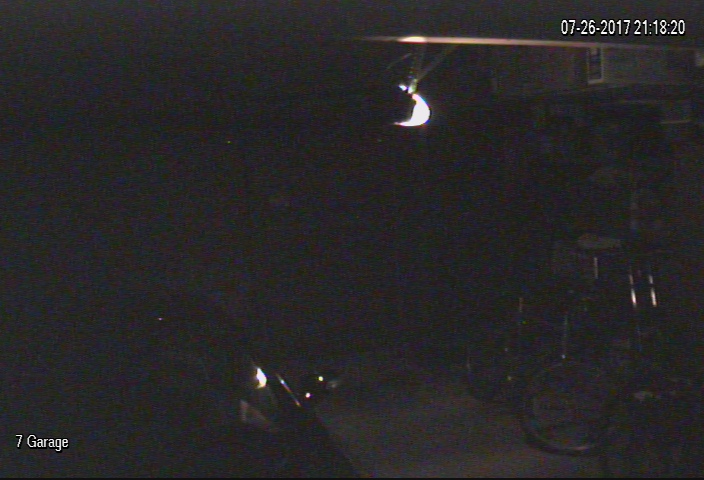Security camera footage captured on July 26th, 2017 at 21:18:20 shows the dimly lit interior of a garage labeled "Seven Garage" in white font at the corner of the image. The date and time stamp are displayed prominently at the top. A faint, glowing white light seeps through the partially open garage door, slightly illuminating the dark-colored vehicle parked inside. The garage contains several bicycles, visible by two wheels and a seat, as well as shelving units with white storage tubs stacked on top. The overall graininess and low lighting of the image obscure further details.